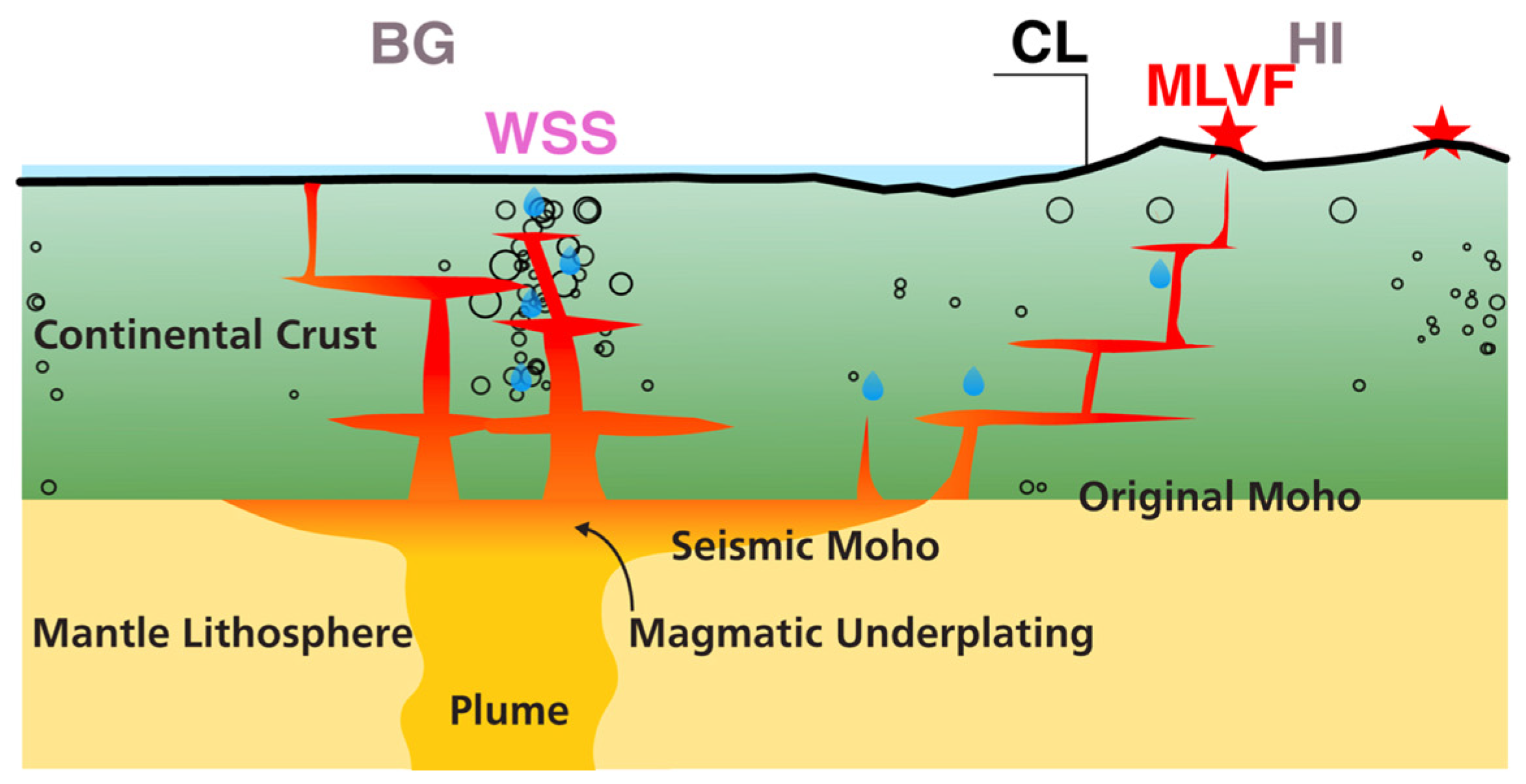The image is a detailed scientific diagram, commonly seen in educational settings, illustrating the structure beneath the Earth's surface. The diagram has a vertical split down the middle, featuring different strata. The top portion displays a body of water extending about three-fourths across, with bubbles visible just below the surface. Beneath this, the green-labeled "continental crust" stretches across, gradually transitioning into yellow, orange, and red hues as it descends, representing mantel lithosphere, mantle, and magmatic features. 

Notably, a stair-like formation shows magma or lava ascending towards the surface, pushing through the continental crust. Key labels include mantle lithosphere, seismic Moho, original Moho, and magmatic underplating. The diagram meticulously maps out the internal flow of Earth's materials, highlighting an orange plume rising from the deeper layers. This visually striking illustration cross-sections the geological processes, from sub-surface magmatic activity to interactions at the continental crust, vividly depicting Earth's dynamic interior architecture.